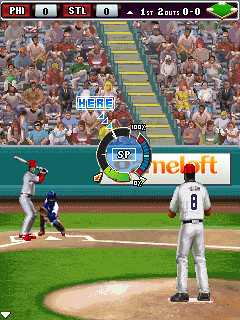A digital screenshot from a baseball video game captures a dynamic scene at the pitcher's mound. The foreground to the right features the pitcher's mound, a distinctive brown dirt circle. Centered on the mound is the pitcher, identifiable by his white uniform and red hat. His dark skin contrasts with the white and red of his attire. He stands poised on a white rectangle, his black cleats solidly planted, with a blue number 8 prominently displayed on the back of his jersey. Surrounding the mound is a vibrant grassy field.

In the batter's box stands a batter dressed in a gray jersey and pants, paired with red shoes and a red helmet. He grips the bat backward, readying for the pitch. To the left, the catcher, outfitted in a blue face mask and matching body gear, is crouched, leaning slightly to his left in anticipation of the pitch. 

Behind the players, a crowd is visible, separated by a blue barrier, adding depth and atmosphere to the scene. At the center of the screen, a pitching indicator reads "100% SP." The game's scoreboard at the top edge shows PHI 0, STL 0, with a count of 0-0, two outs, and no runners on base.